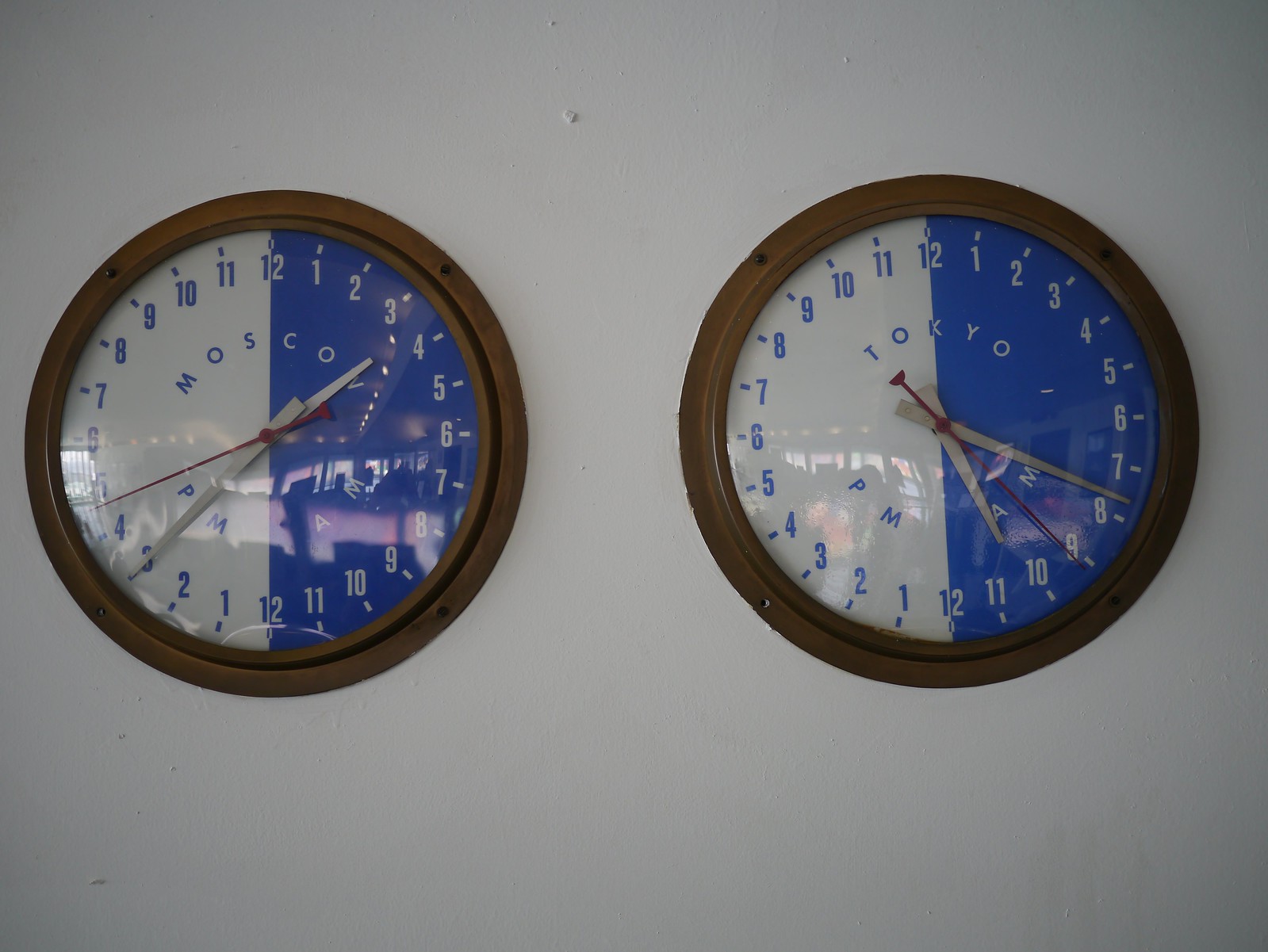In this color photograph, a gray wall serves as the background for two circular clocks mounted side by side. The clocks are encased in brown plastic rims and feature a unique blue-and-white design. The clock on the left is labeled "Moscow" and is divided into two distinct halves: the right half has a royal blue background with white numerals ranging from 12 to 12, while the left half displays a white background with blue numerals ranging from 1 to 11. The minute and hour hands are silver, and the second hand is red. The clock on the right follows the same design, labeled "Tokyo" and displays AM to PM. Both clocks share the same color scheme and hand designs, providing a vibrant yet functional display of time zones.